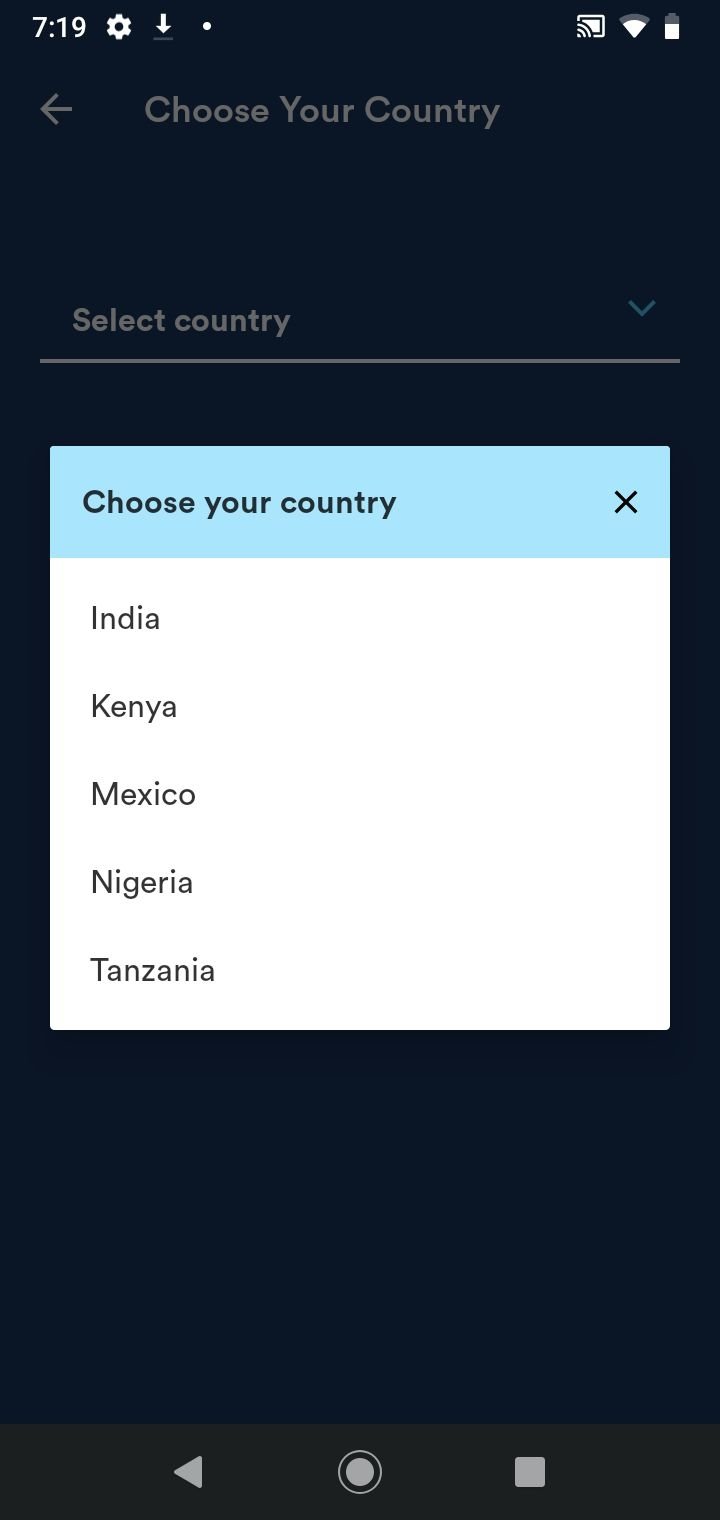A digital screen displays the number "719" which appears to be associated with an item or selection. At the top of the interface, there is an option labeled "Choose Your Country," accompanied by a left-pointing arrow. Below, the text "Select Country" is prominently displayed within a light blue rectangle, featuring the phrase "Choose Your Country" in black font. There is also a close button (X) for exiting this selection menu. The list of available countries includes India, Kenya, Mexico, Nigeria, and Tanzania. At the bottom of the screen, a black rectangle contains white symbols: a left-pointing arrow, a circle, and a square, likely indicative of navigation or input options.